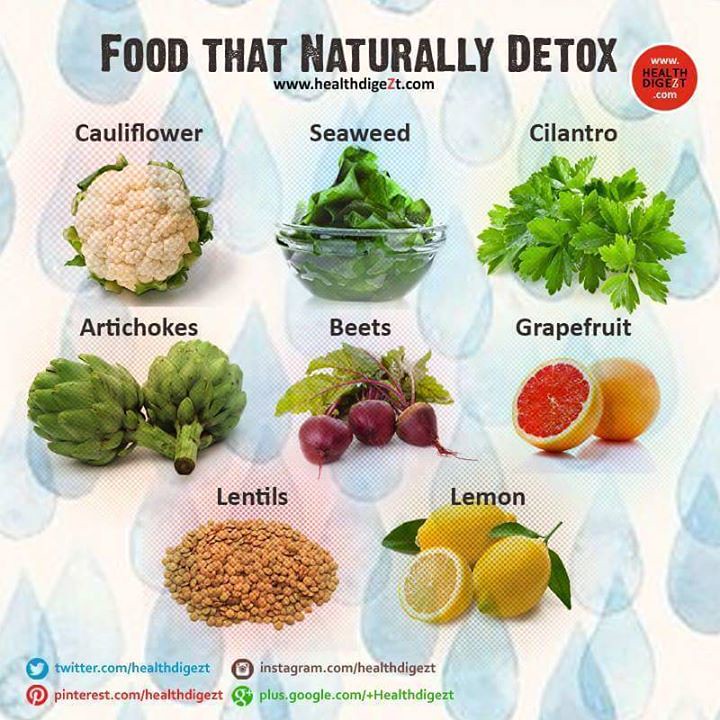The poster titled "Food that Naturally Detox" has a white background adorned with subtle blue water drops. At the very top, "www.healthdigest.com" is prominently displayed. Additionally, there's a red sticker to the right that repeats "www.healthydigest.com." The poster features a neatly organized list of detoxifying foods accompanied by their images, arranged in rows. The first row showcases cauliflower, seaweed, and cilantro. The second row begins with two artichokes, followed by three beets with their leaves, a whole grapefruit, and a grapefruit cut in half. The third row includes an oval-shaped pile of lentils and concludes with two whole lemons with green leaves, alongside a lemon cut in half. In the bottom left corner, links to Healthy Digest's social media profiles on Twitter, Instagram, Google Plus, and Pinterest are noted.